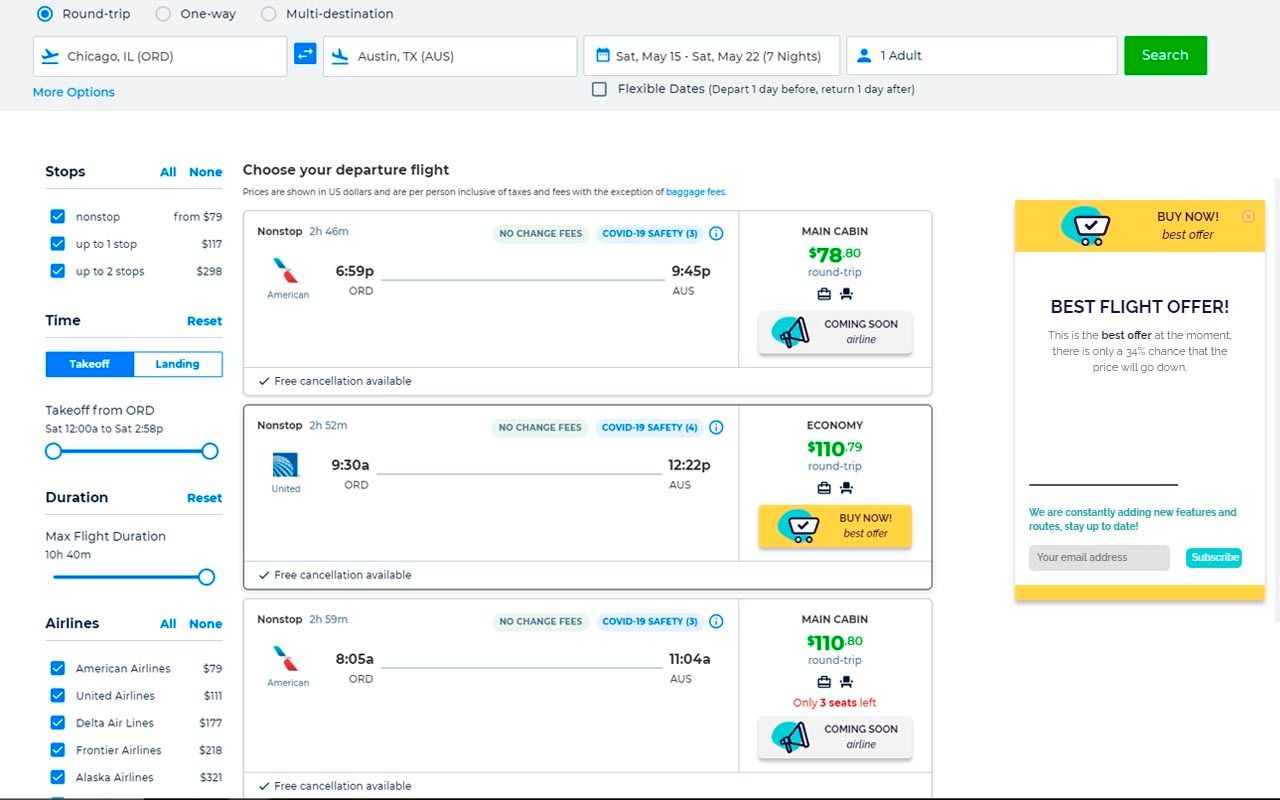This image is a detailed screenshot of a flight booking website displayed against a white background. The top of the page features a light gray border, containing options for different trip types: "Roundtrip," "One-Way," and "Multi-Destination." The "Roundtrip" option is currently selected, highlighted in blue.

Below the trip type, there is a row of four text boxes. The first box shows the departure city as "Chicago, Illinois," and the second one displays the arrival city as "Austin, Texas." The third box includes travel dates, listed as "Saturday, May 15th through Saturday, May 22nd," indicating a seven-night stay. The fourth and final box specifies the number of travelers, showing "One Adult." To the right of this section is a green button labeled "Search."

Beneath this top section, the background remains white. A column on the left side of the page allows users to refine their search based on the number of stops, preferred departure times, maximum flight duration, and chosen airlines.

In the main content area, users are prompted to select their departure flight from three listed options. These options are presented in three separate boxes, each detailing a different flight choice:
1. Non-Stop Main Cabin for $788.00 roundtrip.
2. Non-Stop Economy for $110.00 roundtrip.
3. Non-Stop Main Cabin for $110.00 roundtrip.

On the right side of the page, there's a section titled "Best Flight Offer." This area highlights the second option—Non-Stop Economy for $110.00 roundtrip—as the best current offer. It also informs users that there's only a 34% chance that this price will decrease.